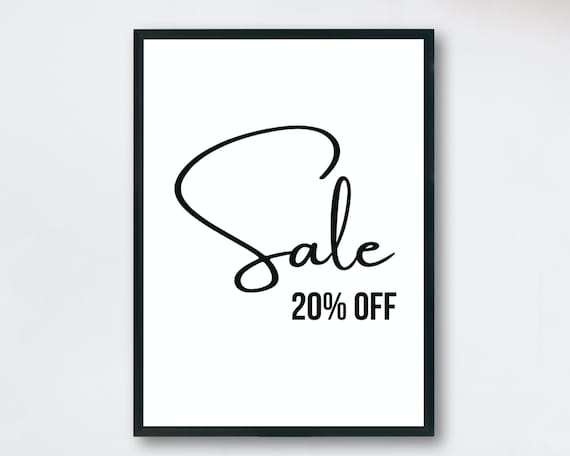In a well-lit image taken with high-quality camera equipment, we see a simplistic and minimalistic setup featuring a black-framed photo hanging on a stark white wall. Central to this gallery-style representation is the word "SALE" rendered in large, swooping cursive script with a very dramatic 'S' that almost defies recognition but is understood from the context. Directly underneath, in a plain typeface font, the words "20% OFF" are inscribed, making the message clear. This framed piece, set against a clear-to-white background, looks more like a front-page advertisement or a digital representation rather than an actual retail object. Its minimalistic appearance, without any other surrounding elements, suggests an abstract commentary on consumerism and retail promotions. This setup resembles an Etsy store presentation rather than an in-store display, further emphasizing its artistic and thought-provoking nature.